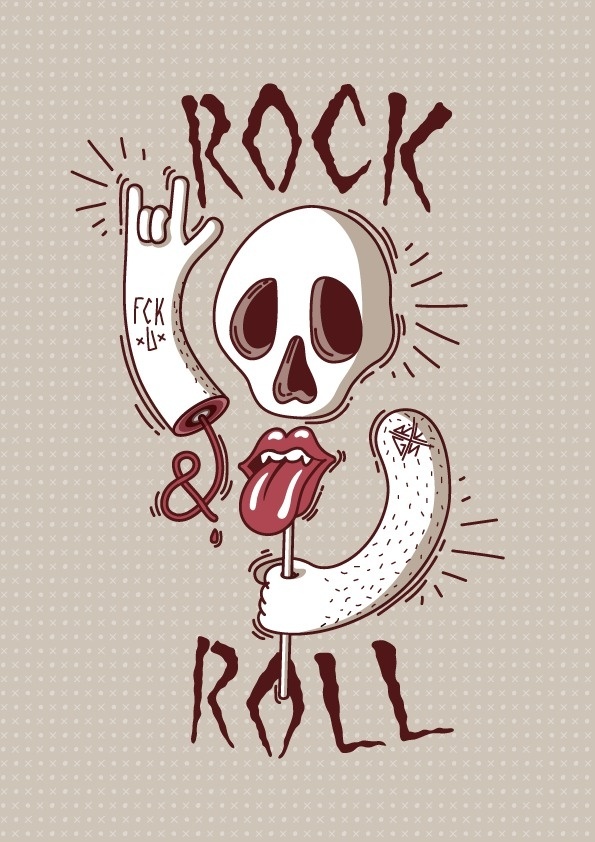The image is a vibrant, hand-drawn graphic with a tan background, intricately patterned with alternating small white X's and O's. Dominating the forefront is a half skull, missing its lower jaw, with hollow, pear-shaped eye sockets and an upside-down heart-shaped nasal cavity, both filled with a burgundy hue. The skull features various lines on its right side, enhancing its detailed appearance. Flanking the skull are two disembodied, floating arms. The arm to the left curves upward, displaying the rock and roll hand gesture, with the index and pinky fingers raised and the thumb extended. This arm has a provocative tattoo reading "FCKU," flanked by X's on either side. The right arm clutches a stick that culminates in the iconic Rolling Stones lips and tongue logo, serving as a mouthpiece. Completing the illustration are the words "rock" at the top and "roll" at the bottom, rendered in bold black text, with an ampersand symbol formed by a bloodline or vein from a cut on the arm. The overall design exudes a gritty, punk rock aesthetic.